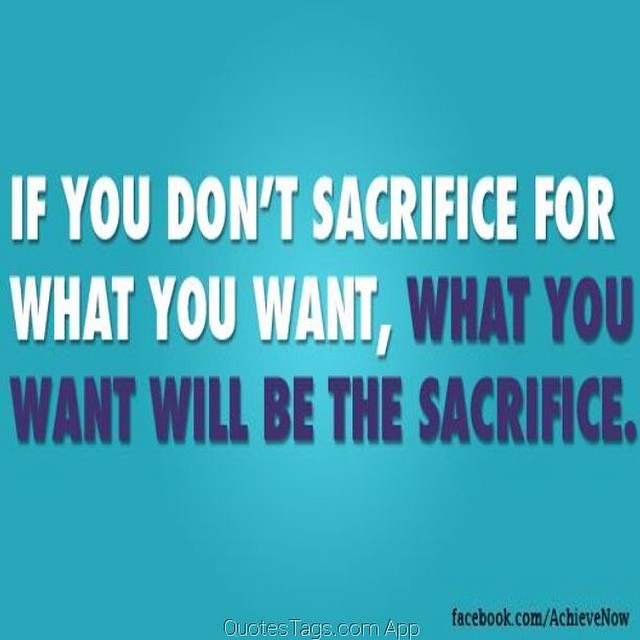This square image features a gradient aqua blue background that darkens towards the edges, becoming progressively lighter as it approaches the center. Prominently starting about a third of the way down from the left-hand side, a motivational quote is displayed: "If you don't sacrifice for what you want," in bold white text, followed by, "what you want will be the sacrifice," in bold navy blue text. At the bottom center, in small, shadowed white or light blue print, is the text "quotes tags dot-com and then app." In the lower right-hand corner, "facebook.com/achieve now" appears in small black print, though slightly blurred, indicating the image might be a photograph of a screen or an enlarged screenshot.